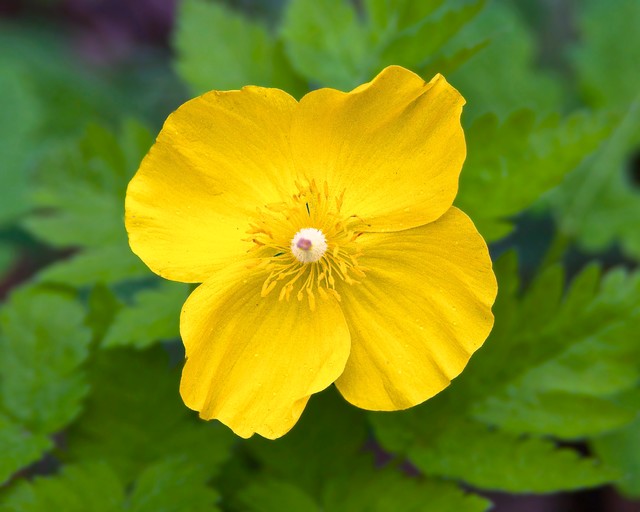The outdoor daytime photograph captures a vivid and healthy bright yellow flower in sharp, crisp focus. The close-up shot, looking down on the flower, highlights its four slightly curved, overlapping petals, each detailed with lines. The round center of the flower prominently displays about 20 to 30 pollen strands and a striking dot that is white with a small pink center. The background features long, green leaves that appear to be fern-like, but these are slightly blurred, creating a contrast that makes the flower pop out almost in a 3D effect. The blurred greenery occupies the majority of the remaining space in the image, emphasizing the central focus on the vibrant bloom. No text or lettering is present on the photograph.